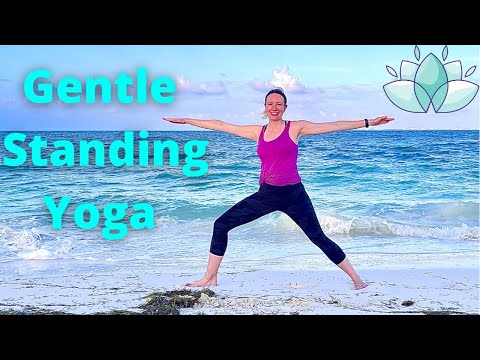The image is a detailed screenshot of a YouTube video thumbnail titled "Gentle Standing Yoga." It features a white-complexioned woman with dark brown hair tied in a ponytail, standing in a yoga pose on a sandy beach during the daytime. She wears a maroon tank top, black yoga pants that extend halfway down her knee, and a fitness tracker on her left wrist. The woman’s arms are outstretched horizontally, with her left leg straight and her right knee slightly bent, leaning into her right leg. A serene ocean with slight waves and a backdrop of blue sky and clouds can be seen behind her, along with some seaweed on the beach to her left. She appears to be smiling and slightly red in the face, looking directly at the camera. The thumbnail has black bars at the top and bottom with text and design elements, including a blue-green caption reading "Gentle Standing Yoga" and a light and dark blue-green lotus flower emblem in the upper right corner. The overall color scheme includes a lot of blues and grays, contributing to a tranquil, beachside ambiance.